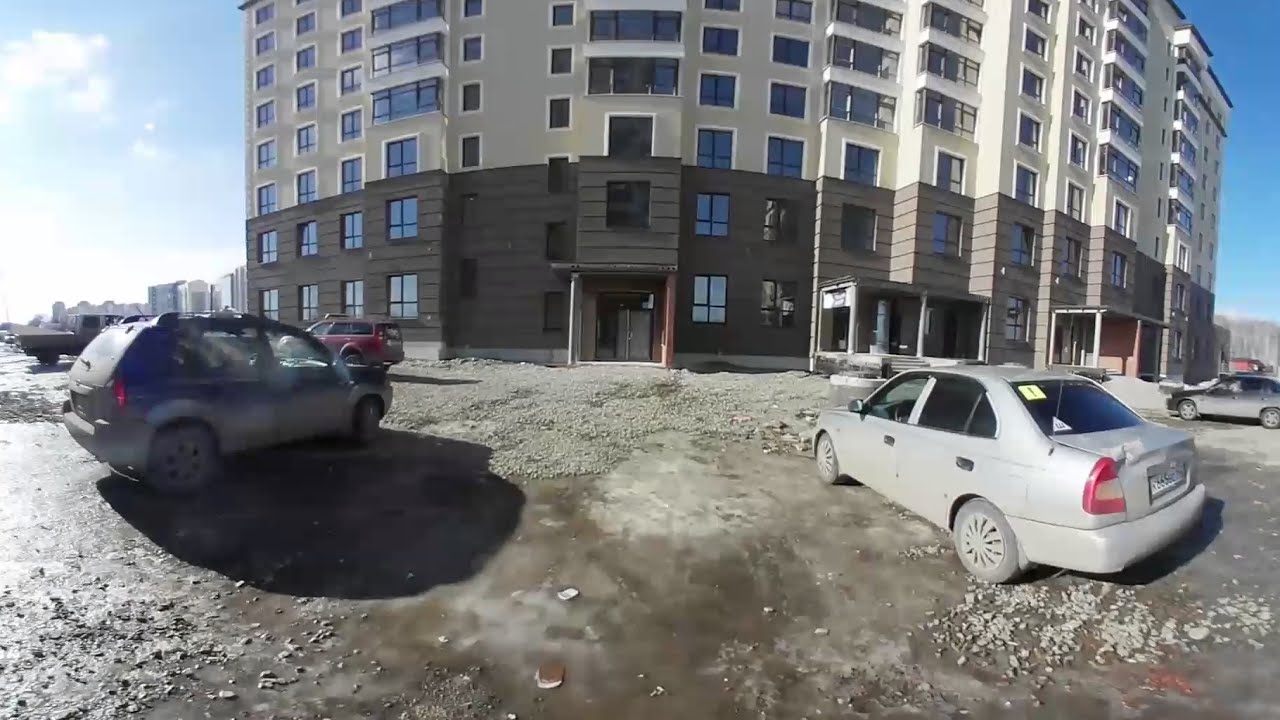The image depicts an outdoor scene featuring a multi-story apartment building with approximately eight floors. The lower two floors of the building are painted a dark brown, while the upper six floors are a lighter beige. Surrounding the building is a parking area, characterized by a mix of gravel, dirt, and partial cement, with some scattered water puddles. In the foreground, a silver or gray four-door car is parked on the right side, its driver and back passenger side door handles highlighted in black. The car has a gold sticker in the upper left corner of the rear glass and a triangular sticker in the bottom left corner. Next to it, a red-colored car and a dark-colored car are also parked. Additional buildings and more parked cars are visible in the background. The sky above is blue, adorned with scattered clouds. Shadows cast by the sun can be seen on the ground, particularly to the right side of an SUV positioned on the left side of the image.